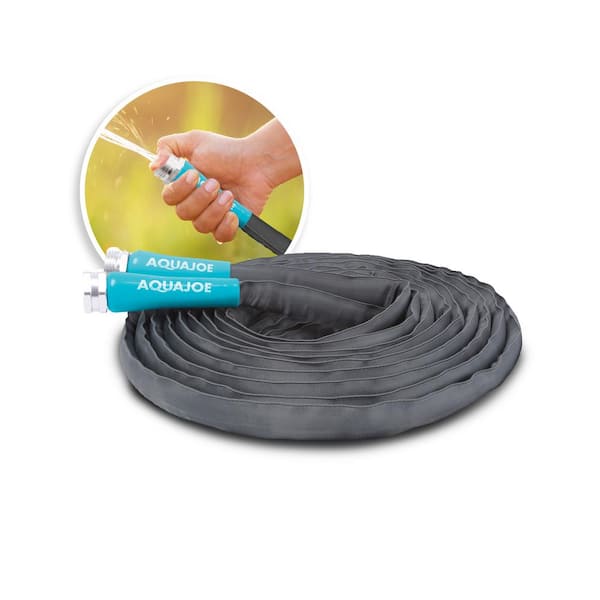This image appears to be an advertisement set against a simple white background, featuring a black water hose that is neatly coiled. The coiled hose has aqua-colored tips with silver caps, and the brand name "Aqua Joe" is prominently displayed in white lettering on each end of the hose. Above the main image, there is an inset circular picture showcasing a close-up of a Caucasian hand holding the hose, using a thumb to partially obstruct the flow, causing water to spray out forcefully. The hose is described as having a soft, expandable material that lies flat when not in use. The overall composition effectively highlights the hose's design and functionality, suggesting its use for tasks like washing a car where controlled water pressure is beneficial.